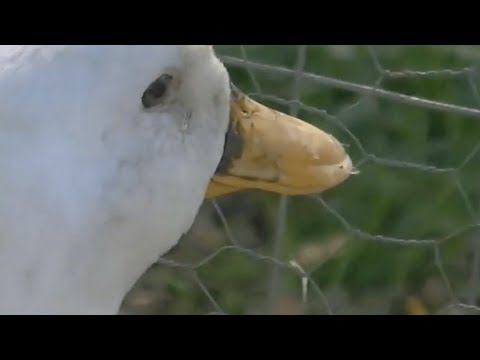The close-up image captures the head of a duck with a white plumage and a yellowish-orange beak. The duck's head is positioned on the left side of the frame, partially facing right towards a chain link fence, with its beak nearly touching the wire. Although the top of the head and most of the neck are not visible, the duck's distinctive features are prominent: its eye, dark with a black center surrounded by lighter feathers, and a dull gray-brown area where the beak meets the face. In the background, slightly blurred, stretches a verdant grassy field. The chain link fence has large hexagonal openings, some of which align right behind the duck's beak and eye. Additionally, the image's upper and lower edges are marked with thick black bands, and there's a hint of sunlight casting a subtle light on the upper left corner of the frame.